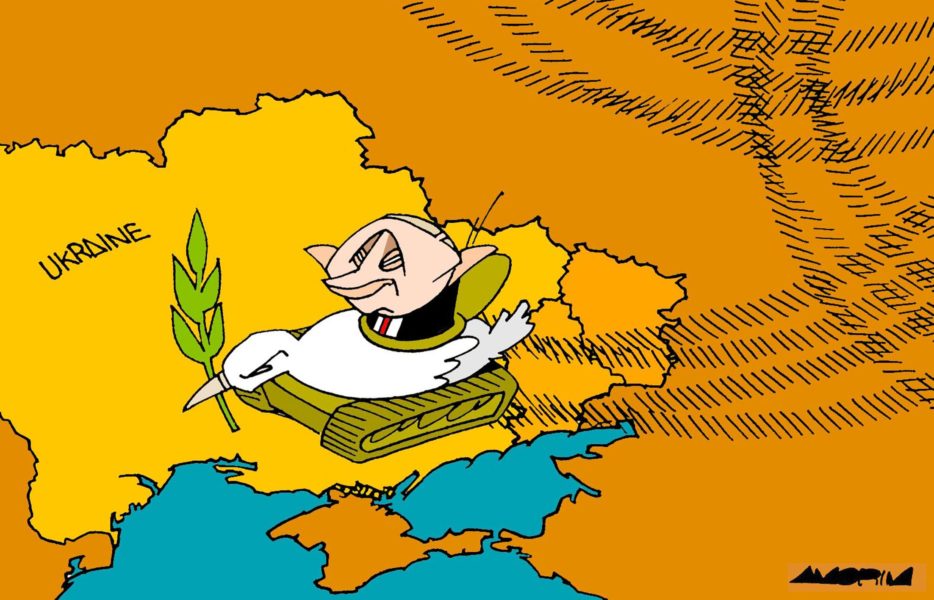This cartoon-like image depicts a caricature of Vladimir Putin riding a green tank, which is moving from Russia into Ukraine. The tank features a white dove carrying an olive branch perched on its front, symbolizing a paradoxical message of peace amidst the military imagery. Putin, dressed in a black suit with a red tie, is seen popping out of the top of the tank. The map background highlights Russia in a dark orange hue and Ukraine in a dark yellow hue. Ukraine's border is marked in black, with the country name spelled out using a distinctive triangle shape in place of the 'A'. Tank tracks illustrate the path from Russia to Ukraine, suggesting repeated incursions. Beneath both countries, a blue ocean is visible. In the lower right corner, there is an indistinct autograph composed of triangular shapes.